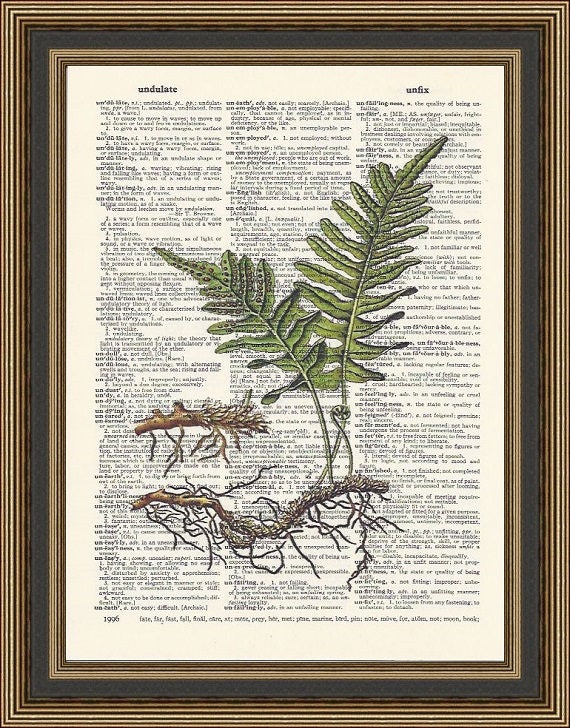This framed artwork features an ornate, green and gold frame enclosing a vintage dictionary page with the words "undulate" and "unfix" visible at the top. Positioned centrally on this somewhat sepia-toned, small-print dictionary page is a detailed botanical specimen: two green fern fronds with multiple smaller leaves and a visible segment of the fern's root system. The roots are brown and exhibit smaller rootlets branching off, bringing a touch of natural complexity to the piece. Additionally, a small seedling emerges from a branch, enhancing the biological aspect of this decorative and scientifically evocative display. Overall, the piece exudes an antiquated charm, blending botanical illustration with literary elegance.